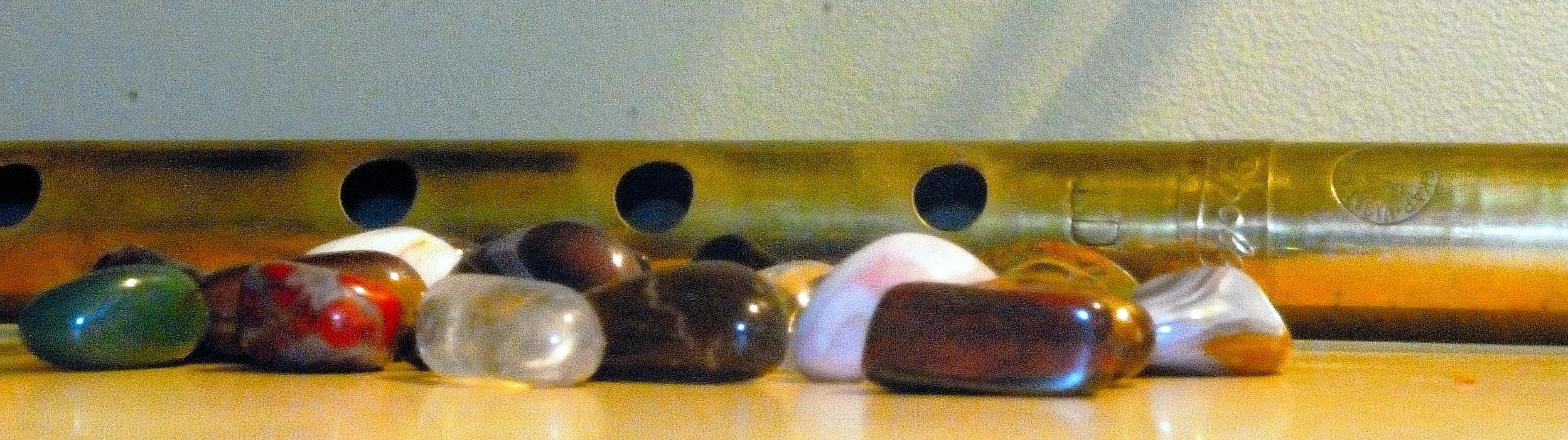The image features an arrangement of 13-14 small, tumbled gemstones, each with oblong spherical shapes, displayed on a light brownish tabletop or desk. The stones are a variety of colors, including green, brown, white, clear, gray, pink, red, and gold, and many possess distinct patterns such as spots or swirls. The gemstones reflect the lighting off the surface of the desk. Behind the stones stands a gold-colored cylindrical object, resembling a metal flute or pipe, marked by four circular holes. This object is set against a white-colored wall, adding depth to the scene. The most prominent stones are a red, orange, and gray one, alongside a notably green one.